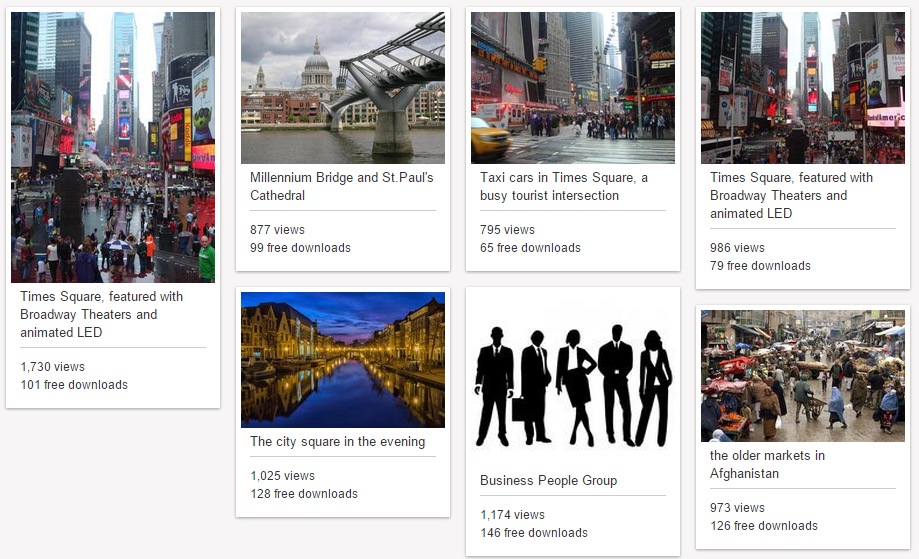**Screenshot of a Webpage with Photo Gallery**

The background of the webpage is gray, adorned with numerous small white squares each containing different photos accompanied by text in black font. 

***Topmost Left Section:***
- **Largest Square:** Displays a vibrant photo of Times Square, New York City. It captures a bustling street filled with tourists, surrounded by towering skyscrapers decorated with dynamic digital billboards. Below the image, the text reads: "Times Square featured with Broadway theaters and animated LED." The photo has "1,730 views" and "101 free downloads."

***Middle Section (To the Right):***
- **Top Row (Left to Right):**
  1. **First Square:** Features an image of a Capitol building set against a serene river with a monorail system spanning across it. The accompanying text is: "Millennium Bridge and St. Paul’s Cathedral." This photo has garnered "877 views" and offers "99 free downloads."
  2. **Second Square:** Shows another view of Times Square, but this time focused more on the street level. It includes a yellow taxi amidst the hustle and bustle. Below the image, it says: "Taxi cars in Times Square. A busy tourist intersection." The photo has "795 views" and "65 free downloads."